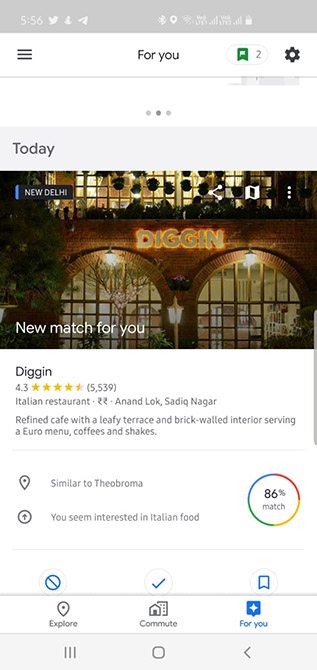**Detailed Caption for the Google Maps Screenshot:**

This screenshot captures a Google Maps page showcasing a restaurant. At the top of the screenshot, there is a white header. On the left, three black lines are stacked vertically, indicating a menu icon. Centered in the header, black text reads "For you." To the right, there is a white, pill-shaped icon outlined in light gray, featuring a green bookmark logo with a white flag icon inside it. Next to the flag icon, the numeral "2" is displayed in medium gray text. Further to the right, there is a dark gray cog icon, likely representing settings.

Beneath the header, the page features a body section with a white background. Near the top, three dots are displayed—the outer two in light gray and the center dot in medium gray. Underneath, a light gray header with dark gray text reads "Today."

The main photo shows a brick building with arched windows. At the center of the photo, a gradient gray logo with a fiery appearance displays the text "Dig In." In the top left corner of the image, a black tag with a blue line on the left side contains white text that reads "New Delhi." The bottom left corner of the photo features white text saying "New match for you."

Continuing below the image, the body of the page returns to a white background. On the top left, gray text reads "Dig In," followed by a light gray rating of "4.3" and four and a half gold stars out of five gray stars. To the right, the number of reviews in parentheses, "(5539)," is indicated in light gray text. Underneath, the category "Italian restaurant" is displayed, followed by a small dot, two rupee symbols, another dot, and the location "Anand Lak, Sadiq Nagar." Lastly, a brief description in the same light gray text style reads, "Refined cafe with a leafy terrace and brick-walled interior serving a Euro menu, coffees, and shakes."